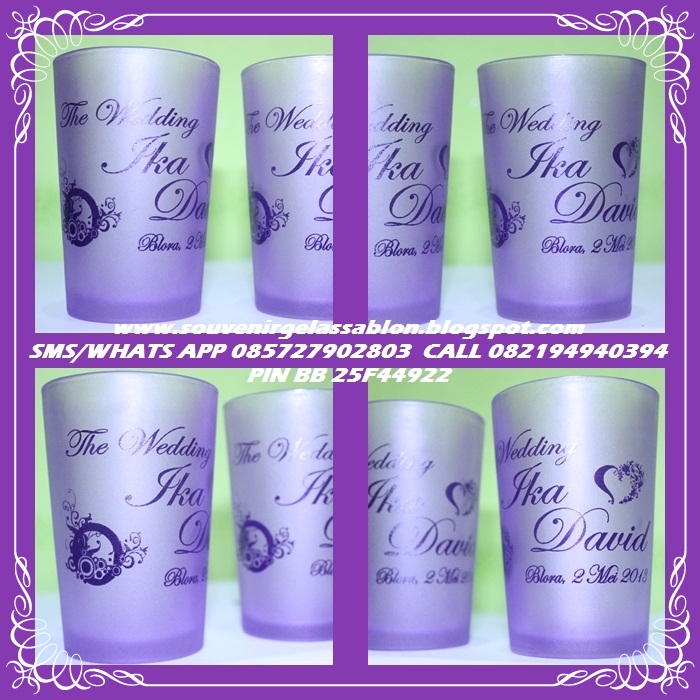This image is a computerized advertisement with a purple background and an intricate white, scroll-like border. It is divided into four sections, resembling window panes with a light green background inside each pane. Displayed within these sections are seven frosted purple shot glasses, each customized with cursive text. The glasses prominently feature phrases such as "The Wedding of" and the names "Ica" and "David," along with heart shapes and likely a wedding date. This ad advertises customizable wedding shot glasses and provides various contact details, including a conspicuous email address, "www.souvenirjesslassonbond.blogspot.com," and two phone numbers usable via SMS or WhatsApp: 0857-2790-2803 and 0821-9494-0394.